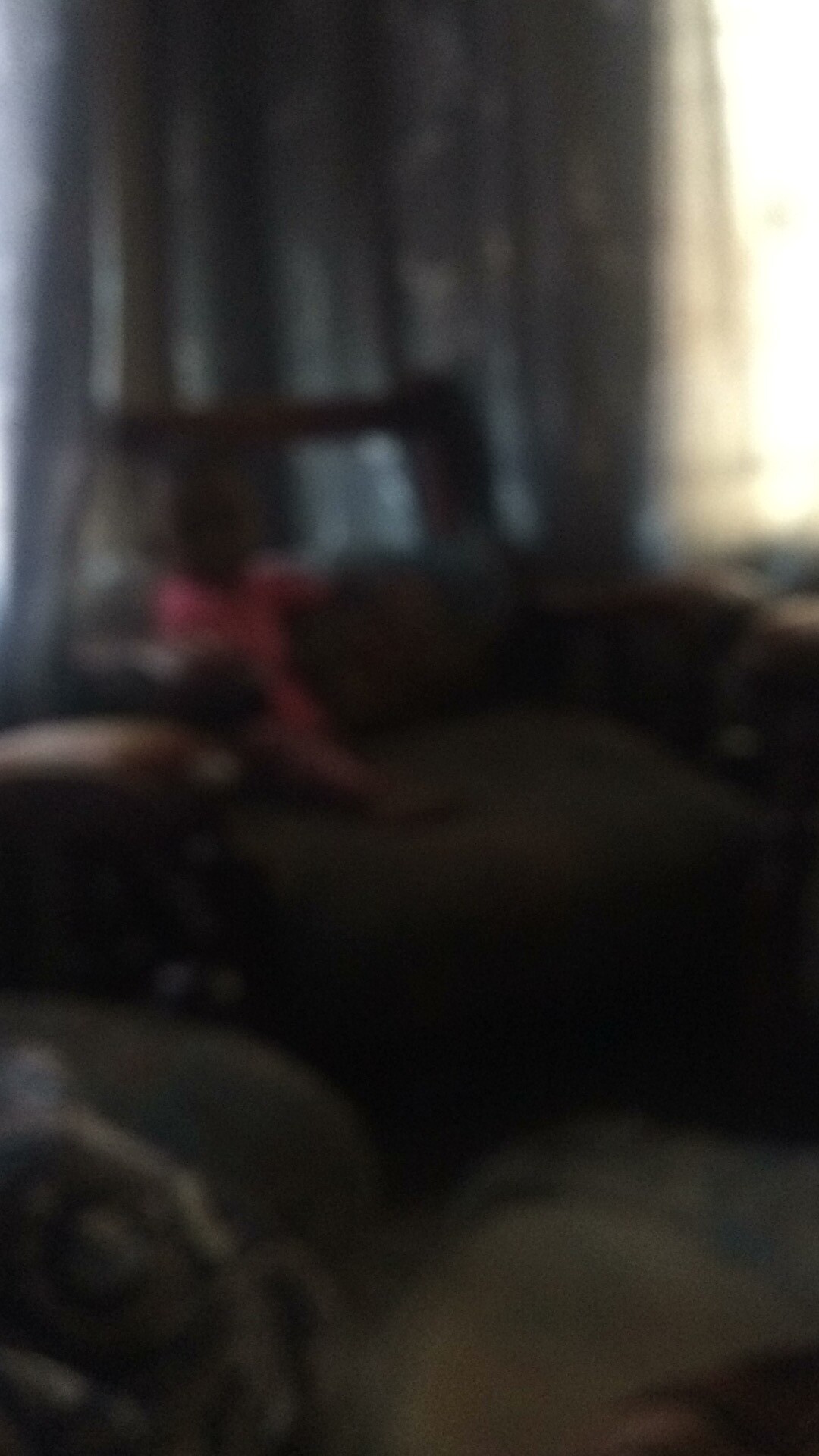This very blurry photograph, presumably taken indoors, captures a dimly lit scene with several indistinct elements. The background features dark-colored, possibly greyish-bluish curtains, with light streaming through a window on the right side, creating a bright contrast in the otherwise dark setting. In the midground, a deep chair—potentially a rocking chair—hosts a small child, who appears to wear a pink outfit, though it's so blurry that details are obscured. Adding to the room's furnishings, there's also a suggestion of a stuffed animal in a red dress on the same chair. The foreground is equally difficult to discern, potentially containing part of a couch or a blanket, with a blur suggesting loose strands of hair. Despite the poor quality of the image, the overall impression is of a cozy, but poorly lit room with a child at its center.